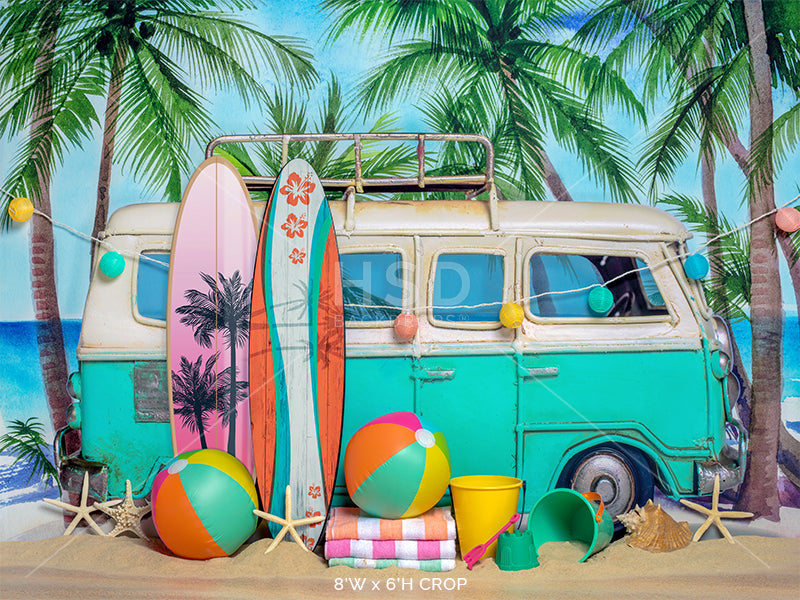This vibrant and detailed image captures a nostalgic beach setting. The scene prominently features a classic turquoise 1968 Volkswagen bus with a cream-colored top, windows up, and two surfboards propped against its side. Surrounding this retro van is an array of lively beach items: two colorful beach balls in hues of green, yellow, orange, and red, and three folded beach towels in striking patterns of yellow and white, pink and white, and green and white. Nearby, there are playful elements like a sand bucket, shovels, a large seashell, and a few starfish scattered on the white sandy ground. Above, a string of lanterns in bright colors (yellow, teal, orange, teal, and pink) stretches between tall coconut palm trees, adding a festive touch. The backdrop boasts a deep blue ocean blending into the expansive sky, completing this picturesque tropical paradise.